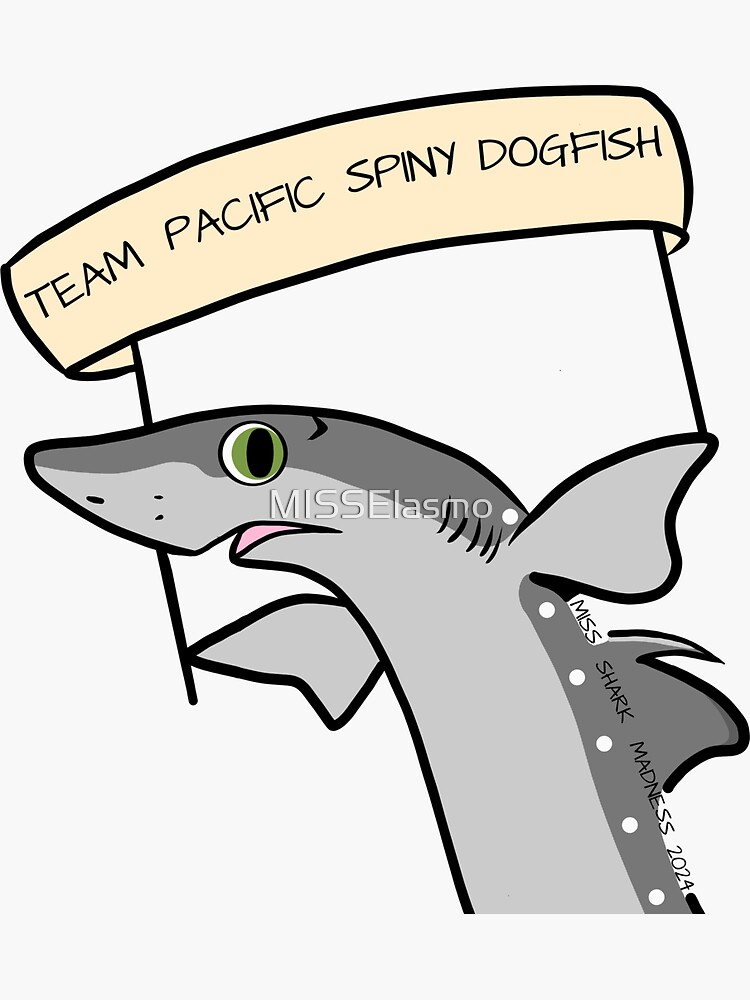This color illustration, in portrait orientation, features a gray shark with distinctive white dots along its dark gray top side and a light gray underbelly. The shark, illustrated from the tip of its nose to mid-stomach, is positioned with its open, pink-mouthed head facing left and body curving towards the bottom right. The shark holds two angled sticks in its side fins, supporting a cream-colored banner that reads "Team Pacific Spiny Dogfish" in black text. The shark's vivid green eye and dark dorsal fin add to its realistic characteristics. A white watermark reading "Miss Elasmo" is emblazoned across its head, while "Miss Shark Madness 2024" is elegantly inscribed along its back. The illustration is set against a light gray background, emphasizing the detailed and striking design.